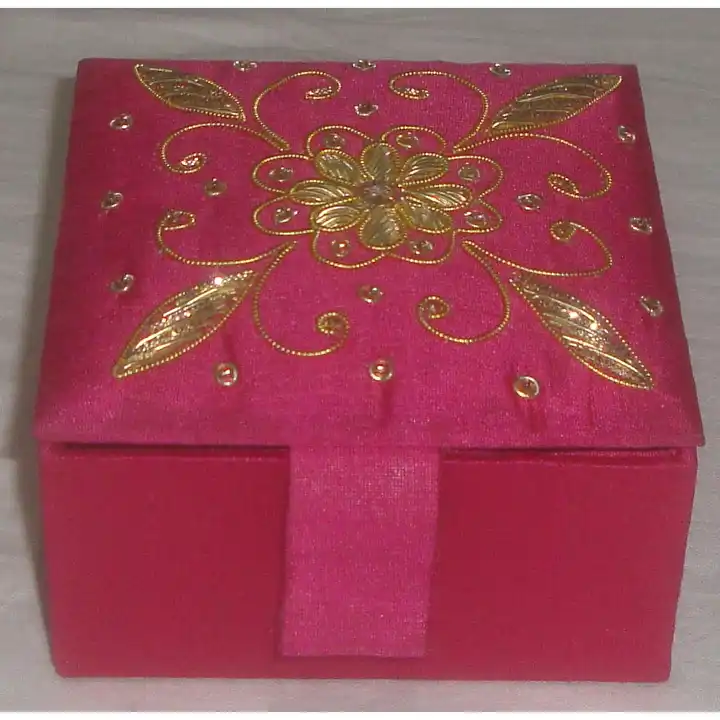Displayed in the image is a small, vibrant bubblegum pink box, portrayed from an above and side angle. The box, which exudes a bold and feminine aura, is set against a gray-toned background, where shadowing is visible to its left. The sides of this very pink box are straightforward and uniform, while the top is adorned with a plush, cloth-covered cushion, offering a soft appearance.

The lid showcases an intricate gold pattern, centralizing on a flower motif embellished with gold beads, resembling sequins. Surrounding the flower are petals, gold-colored swirls, and leaf shapes adding to the ornate design. In each corner of the lid, four additional gold leaves are visible, complementing the central floral pattern. There is a notable pink fabric loop at the front, serving as a handle to lift the lid. The box is slightly ajar, suggesting the functionality of the tab for easy access.